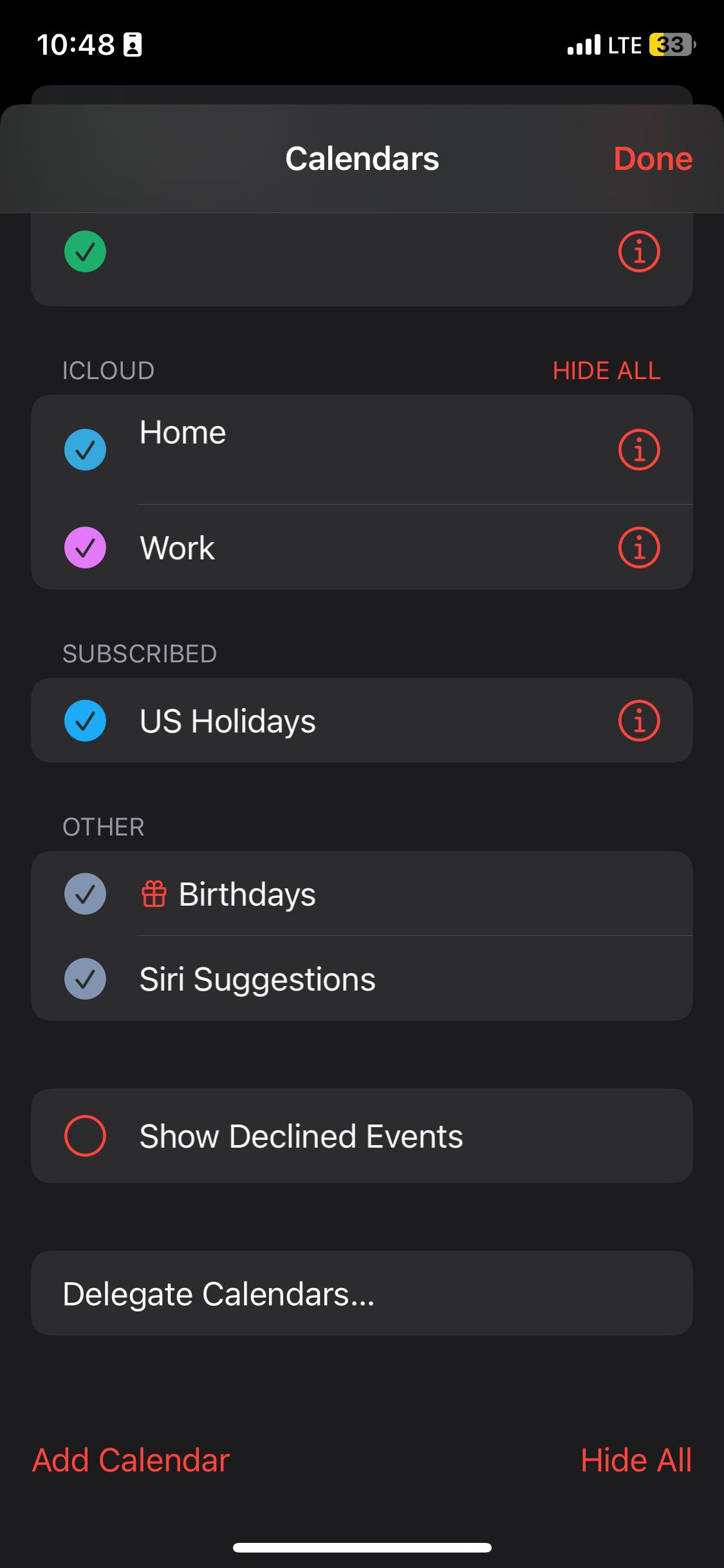This detailed screenshot illustrates a calendar application on an iPhone, confirming its authenticity through visible phone indicators such as the 33% battery life, an LTE network with full coverage (four out of four bars), and the time displayed as 10:48 (AM or PM is unspecified). The interface is set in dark mode, suggesting either the app-specific or the entire phone's mode preference. 

At the top, the calendar app title is nestled within a near-black banner, accompanied by a "Done" button in red at the far right, indicating an actionable option for the user to finalize their entries. Below this, the iCloud section stands out, featuring two selection options—'Home' and 'Work'—both marked active with checkmarks. Adjacent to these checkboxes are small red circles containing the letter 'i,' serving as icons for further information.

Additionally, the screenshot reveals other calendar categories which include 'Subscribed' (specific to US holidays), 'Birthdays,' and 'Siri Suggestions.' This comprehensive setup highlights the user’s organization of personal, professional, and holiday schedules within the digital ecosystem of their iPhone.